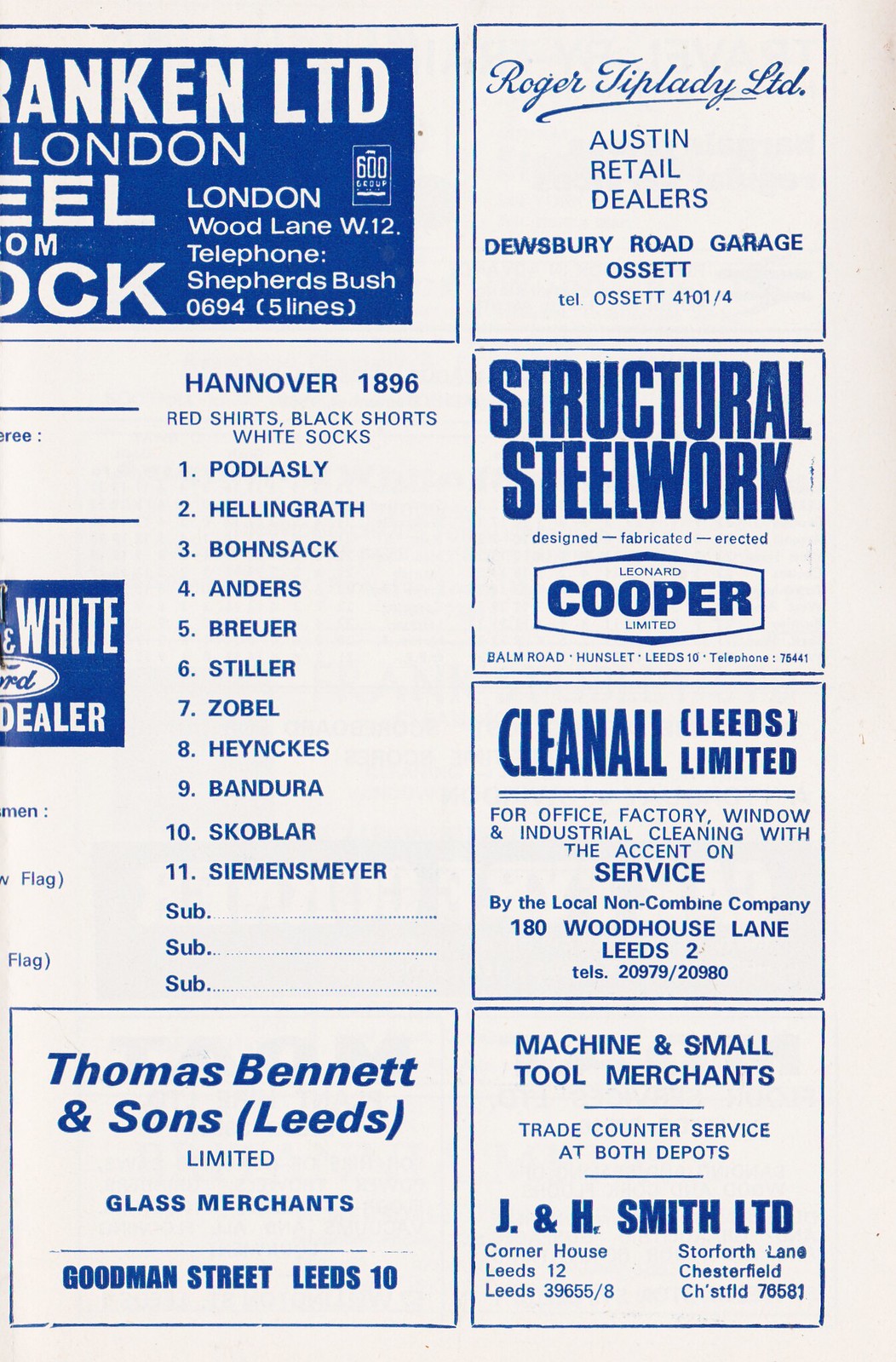A section of a paper placemat is visible, featuring a variety of local advertisements on a white and blue background. Dominating the upper portion is an advertisement for Roger Tiplady Ltd., Austin Retail Dealers, located at Dewsbury Road Garage. Below this is a prominent ad for structural steelwork designed, fabricated, and erected by Cooper Ltd., based on Balm Road, Hunslett, Leeds. Further down is Cleanall Leeds Ltd. offering office, factory, window, and industrial cleaning services, emphasizing their non-combine and local service from 180 Woodhouse Lane, Leeds. J & H Smith Ltd., identified as machine and small tool merchants with trade counter services at depots in both Leeds and Chesterfield, features next. The advertisement section also includes Thomas Bennett & Son, Ltd., glass merchants on Goodman Street, Leeds, and various other brief mentions, like a steel company from Wood Lane, London listed with numerous names suggesting possibly a sports team noting members like Pod, Lasley, Hellingrath, etc.